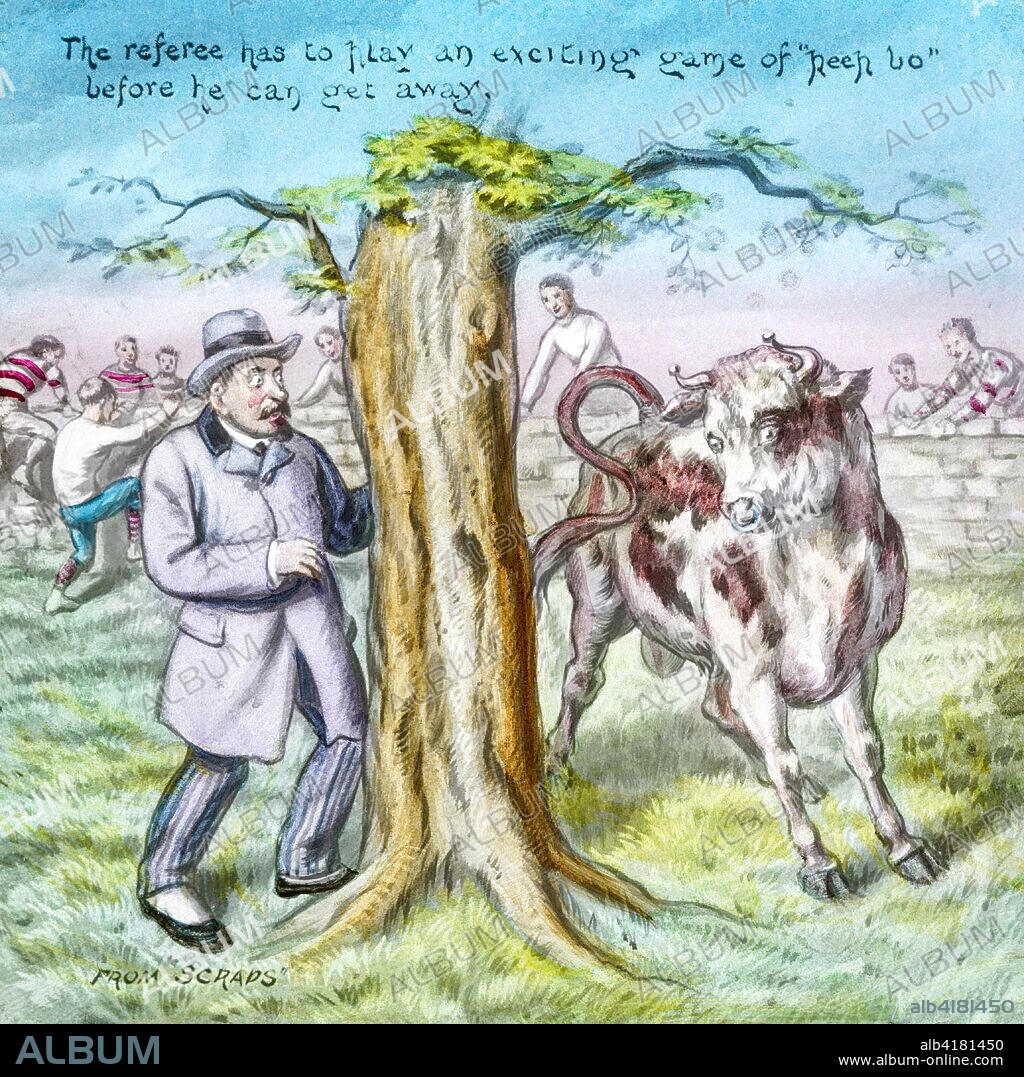The image depicts a quirky, early 20th-century style illustration that blends whimsical and comical elements. At the center, a man dressed in a gray top hat, gray suit, and striped gray and black pants stands on one side of a large tree with exposed roots and green leaves at the top. Opposite him, a white bull with dark reddish patterns, black hooves, and menacing horns appears to be in pursuit. The man’s eyes are wide with surprise, and he sports a mustache, adding to his distinguished yet comical appearance.

In the background, beyond a white brick wall, several figures are depicted mid-action. Some are running away, while others seem to be preparing to climb over the wall or are watching the scene unfold. These figures are dressed in varying outfits, including red and white striped shirts and blue pants, contributing to the chaotic energy of the scene.

Above the central illustration, an inscription reads, "The referee has to lay an exciting game of hee-haw before he can get away." This adds a layer of humorous narrative, suggesting a playful context for the depicted chase. At the bottom left corner, the text "From Scraps" is written, and along the bottom black bar, the words "album" and "www.album.online.com" are faintly visible. The background sky is illustrated with shades of blue and dotted with small white clouds, enhancing the overall whimsical atmosphere of the image.